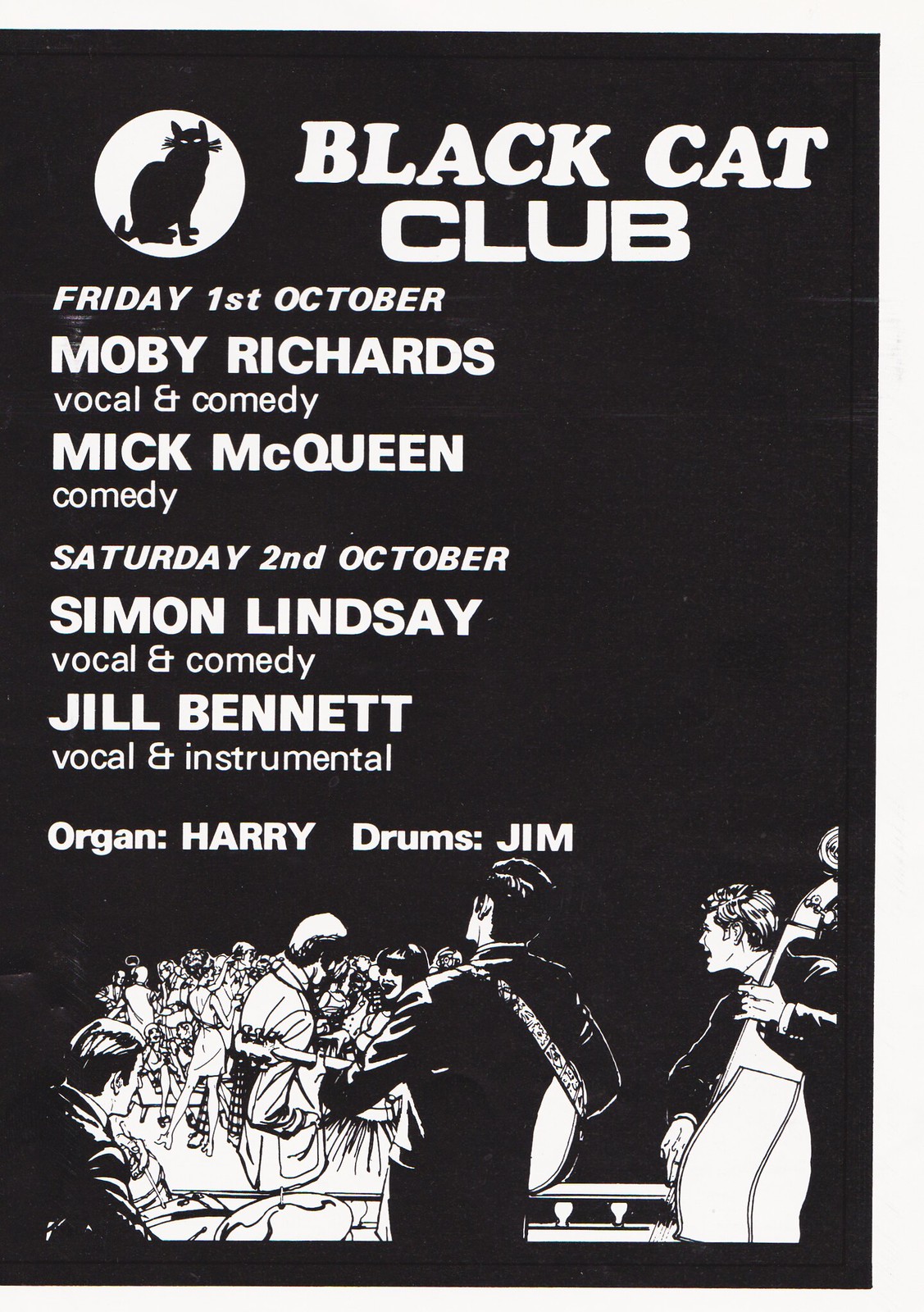The advertisement features a black and white design promoting upcoming live music and comedy events at the Black Cat Club. At the top left, there's a white circle with a silhouette of a black cat with white eyes. Directly to the right, the text reads "Black Cat Club" followed by the event dates and performers: 

- **Friday, 1st October:**
  - Moby Richards (Vocal and Comedy)
  - Mick McQueen (Comedy)

- **Saturday, 2nd October:**
  - Simon Lindsey (Vocal and Comedy)
  - Jill Bennett (Vocal and Instrumental)
  - Organ Harry (Organ)
  - Drums Jim (Drums)

The bottom section of the advertisement showcases a cartoon illustration of a band of three men on stage, performing for a lively crowd. The band members are all dressed in black, with the guitarist in the center, a cellist on the right, and a drummer on the left. The ad combines elements of live music and comedy, underscoring the diverse entertainment offered at the venue. The color scheme of the ad includes shades of black, white, tan, and gray, adding to its striking visual appeal.